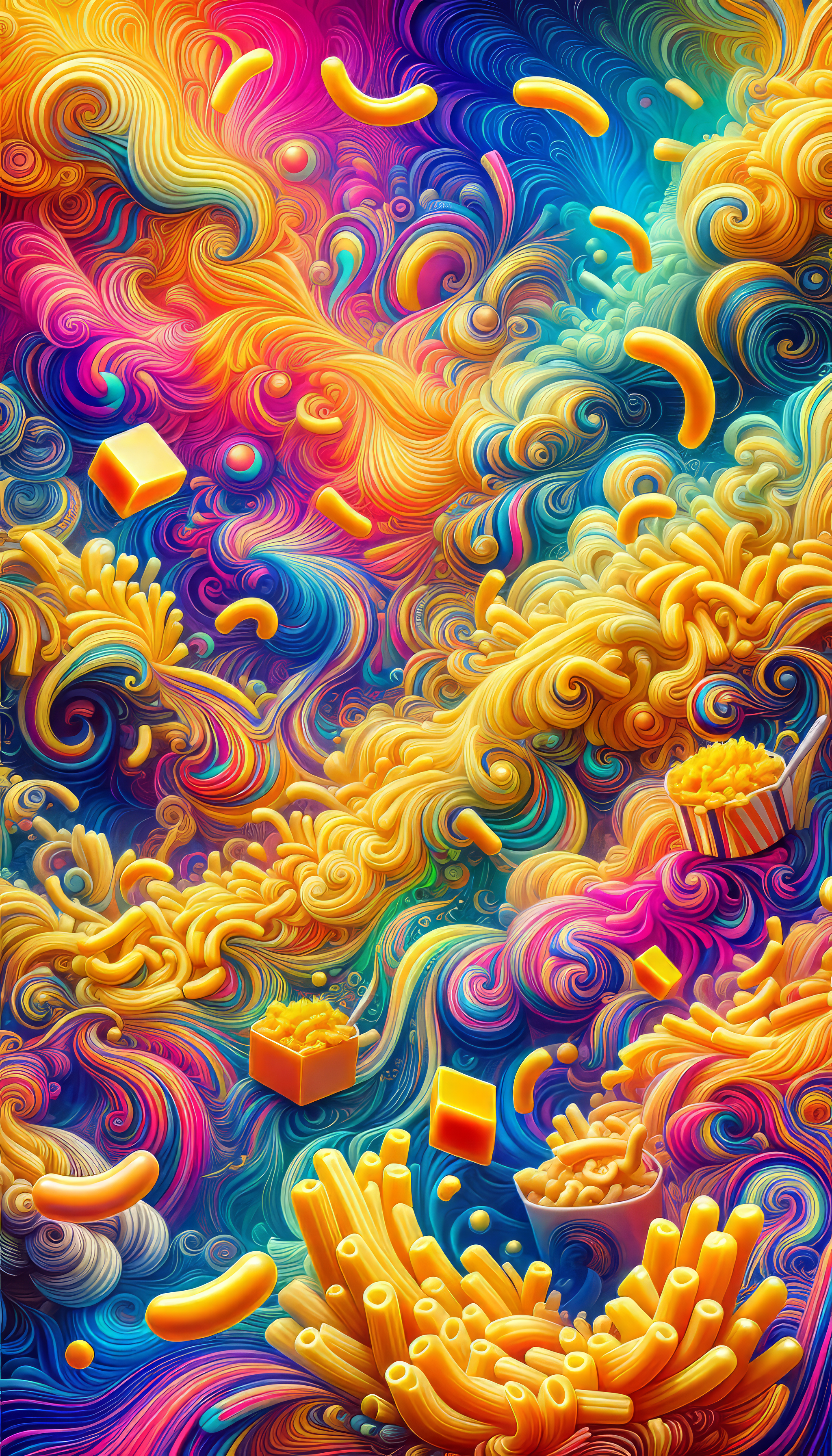The image is a psychedelic and intricate AI-generated artwork featuring a swirling, vibrant array of colors that resemble tie-dye patterns with blues, yellows, greens, and purples blending seamlessly together. The background radiates with these rainbow hues, curling and blurring into each other in little swirls. Interwoven with this colorful chaos are macaroni noodles, rigatoni, and clusters of gooey cheese. Two visible cups of noodles are nestled among the noodles, with one cup more prominent in the front and another slightly obscured in the back. Various cheeses, including some blocky, cube-like pieces, are scattered throughout. A river-like stream of noodles flows down the center, with ribbons of yellow cheese flowing towards the cups. There are also small orange bubbles edged with blue, adding to the dreamy, surreal atmosphere. The image's detailed nature and neon-tinted, paint-like splatters give it an other-worldly, trippy feel, with blocky areas that vaguely resemble macaroni boxes dotting the landscape.